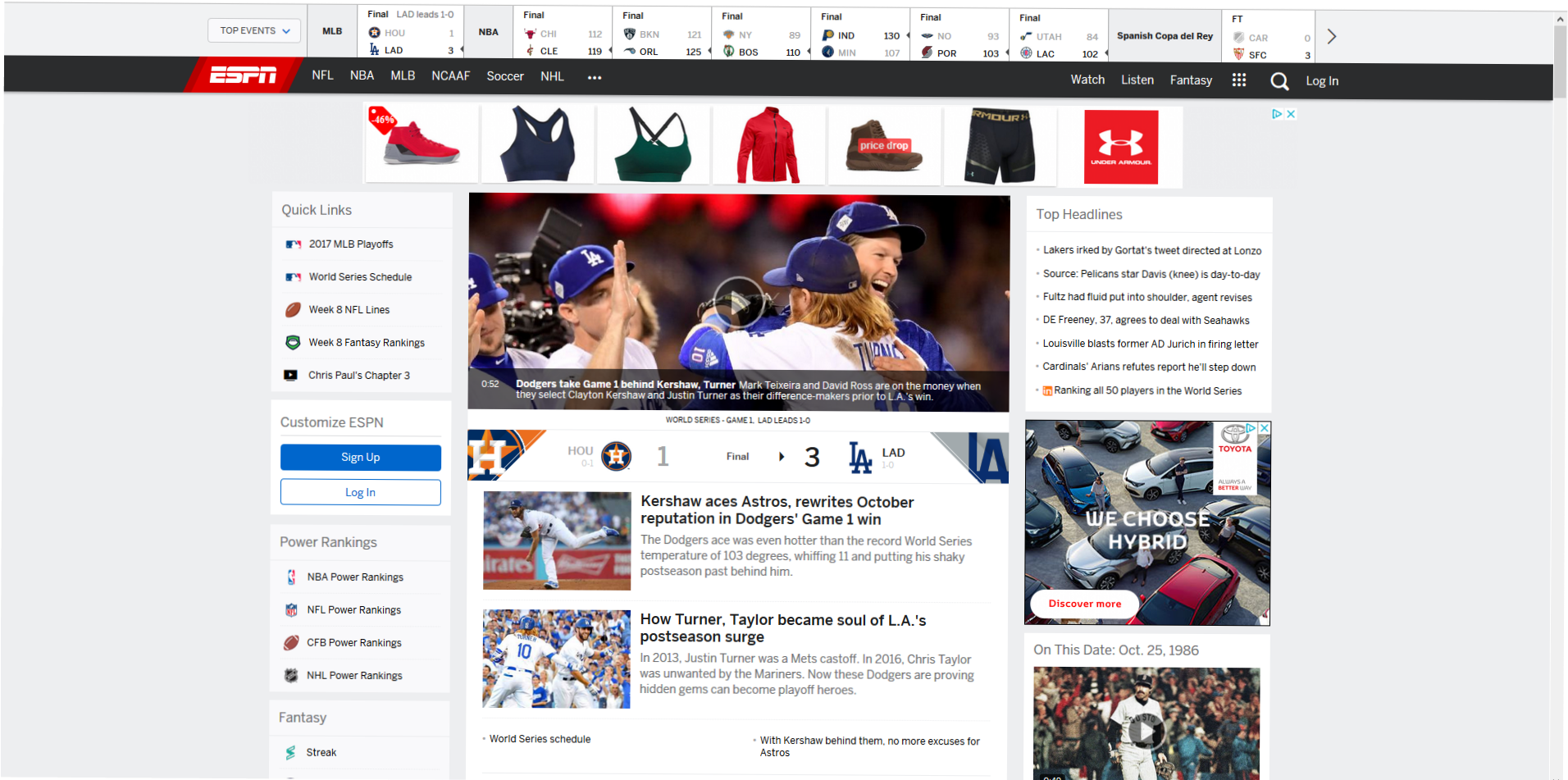The image shows ESPN's website interface. In the upper left corner, there is a dropdown menu labeled "Top Events." Below it, scores from various sports events are displayed, including:

- MLB Final: LAD 3, Honolulu 1
- NBA Finals:
  - CHI 112, CLE 119
  - BKN 121, ORL 125
  - NY 89, VOS 110
  - IND 130, MIN 107
  - NO 93, POR 103
  - UTA 84, LAC 102
- Spanish Cup Del Rey Final: CAR 0, SFC 3

Underneath the events, the ESPN logo appears in white on a red background, followed by a navigation menu with options including NFL, NBA, LVM, NCAAF, Soccer, NHL, and more. On the right side of the page, there are icons and options for "Watch," "Listen," "Fantasy," a nine-dot grid icon, a search icon, and a login button.

Prominently featured is a headline with photographs of LA Dodgers players, accompanied by the text: "Dodgers take Game 1 behind Kershaw, Turner." Analysts Mark Teixeira and David Ross highlight Clayton Kershaw and Justin Turner as key figures in LA's victory.